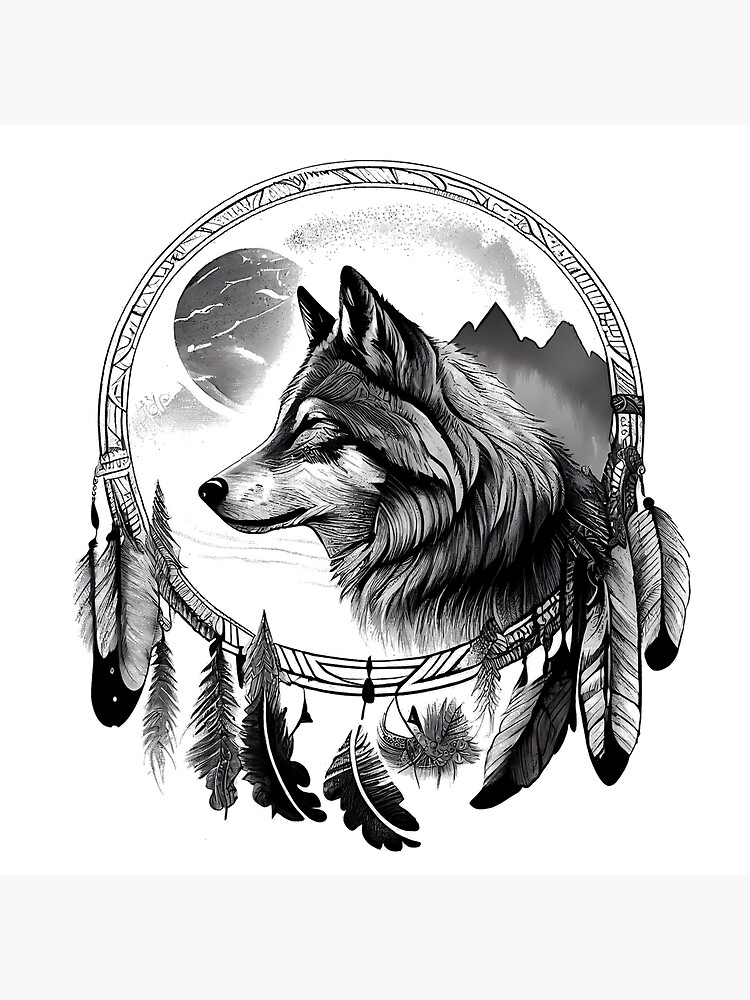This image depicts a striking black, white, and gray dreamcatcher set against a pristine white background. The dreamcatcher features an intricately textured circular frame adorned with artwork. Eleven feathers, attached with leather and decorated with beads, dangle from the bottom of the circle, displaying a mix of black, white, and gray hues. Inside the frame lies a detailed scene where an Arctic wolf, its fur rendered in shades of black, gray, and white, is depicted in profile, gazing to the left with eyes that appear partially closed. Behind the wolf, a rugged mountain range etched with light and dark gray stands, and a celestial body—likely a moon—floats in the sky, described with white lines. The contrast between the detailed elements and the stark white background enhances the ethereal quality of the composition.